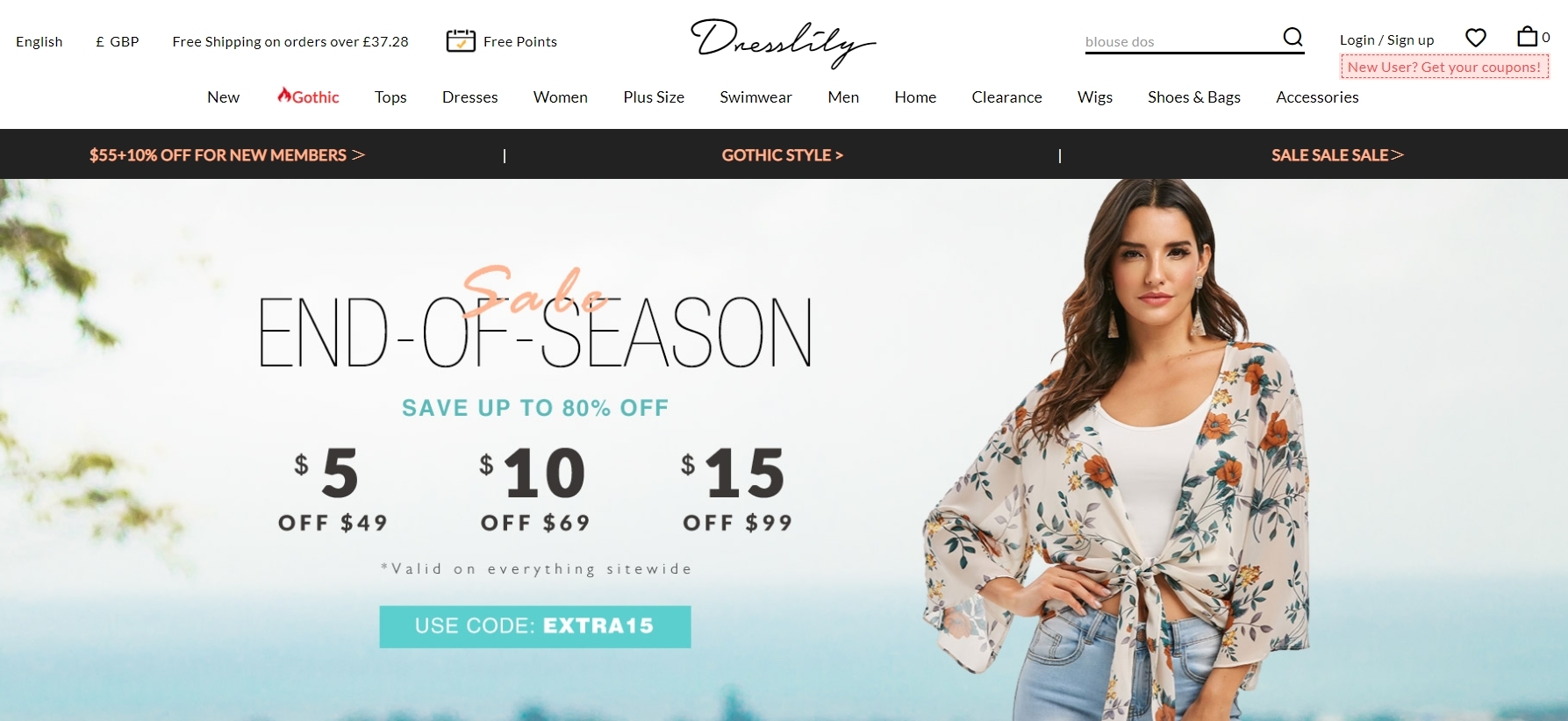This captivating image displays the landing page of Dresslily, an online retail store. At the top of the screen, a plethora of text appears, indicating the site's offerings and promotions. The text, predominantly in English and featuring prices in pounds, highlights several key deals, such as free shipping on orders over £37.28 and the opportunity to earn free points. The header also identifies the platform as Dresslily and showcases various categories including New Gothic Tops, Dresses, Women Plus Size, Swimwear, Men, Home, Clearance, Wigs, Shoes, Bags, and Accessories.

Centrally positioned, a prominent banner advertises a seasonal sale: $5 off orders of $49, $10 off orders of $69, and $15 off orders of $99, applicable site-wide. The promotion encourages customers to use the discount code "EXTRA $15" for additional savings.

The visual centerpiece of the landing page features a woman standing against a scenic coastal backdrop. She is clad in a stylish ensemble consisting of a white tank top layered under a white blouse and a pair of jeans or possibly jean shorts. The model accessorizes her look with drop earrings. To the left side of the photo, distant trees by what appears to be an ocean adds a natural touch to the composition. The serene blue-green hues of the water accentuate the tranquil setting.

Additional promotional text declares, "£55 plus 10% off for new members," and emphasizes recurring sales with exclamatory "Sale, Sale, Sale" messages. The overall design and offers prominently highlight Dresslily's Gothic style collection and other fashion categories.